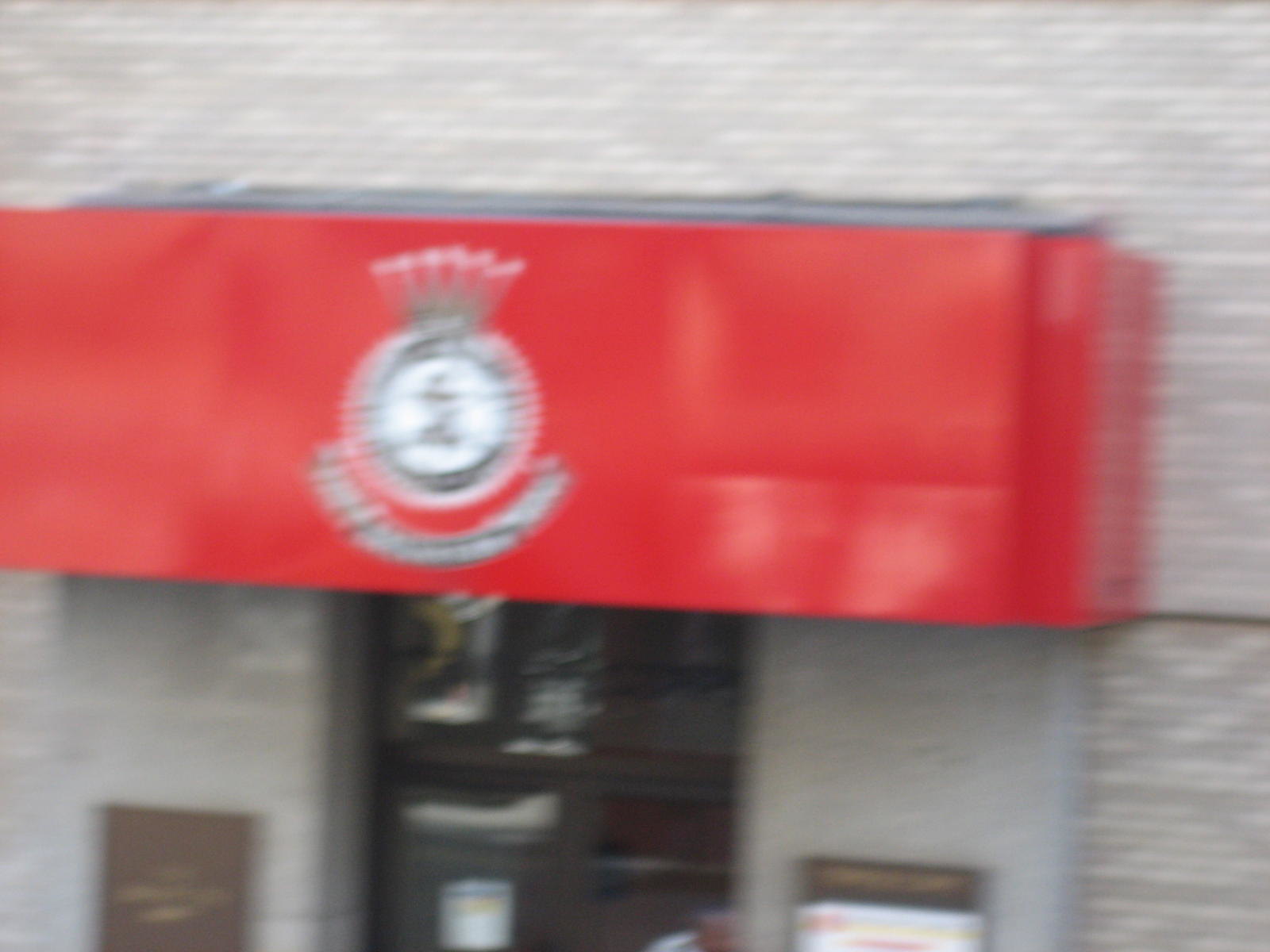This image depicts a very blurry building that resembles a VFW veterans hall or community center. The focal point is a large, prominently placed rectangular red banner that stretches horizontally across the facade, about two inches from the top, extending from near the left edge of the image to about two inches from the right edge. This banner features a central circle design that appears to have crown-like spikes or arrows radiating outward, creating a distinctive emblematic pattern. Below the banner, at the center of the image, is the entrance to the building—a glass door that has several indistinguishable posters due to the blurriness of the photo. The building itself is primarily composed of light gray brick with some portions of concrete and features a small brown square at the bottom of the left side. Additionally, there is a smaller sign in front of the building that is brown on top and white on the bottom, although its details are not clear.